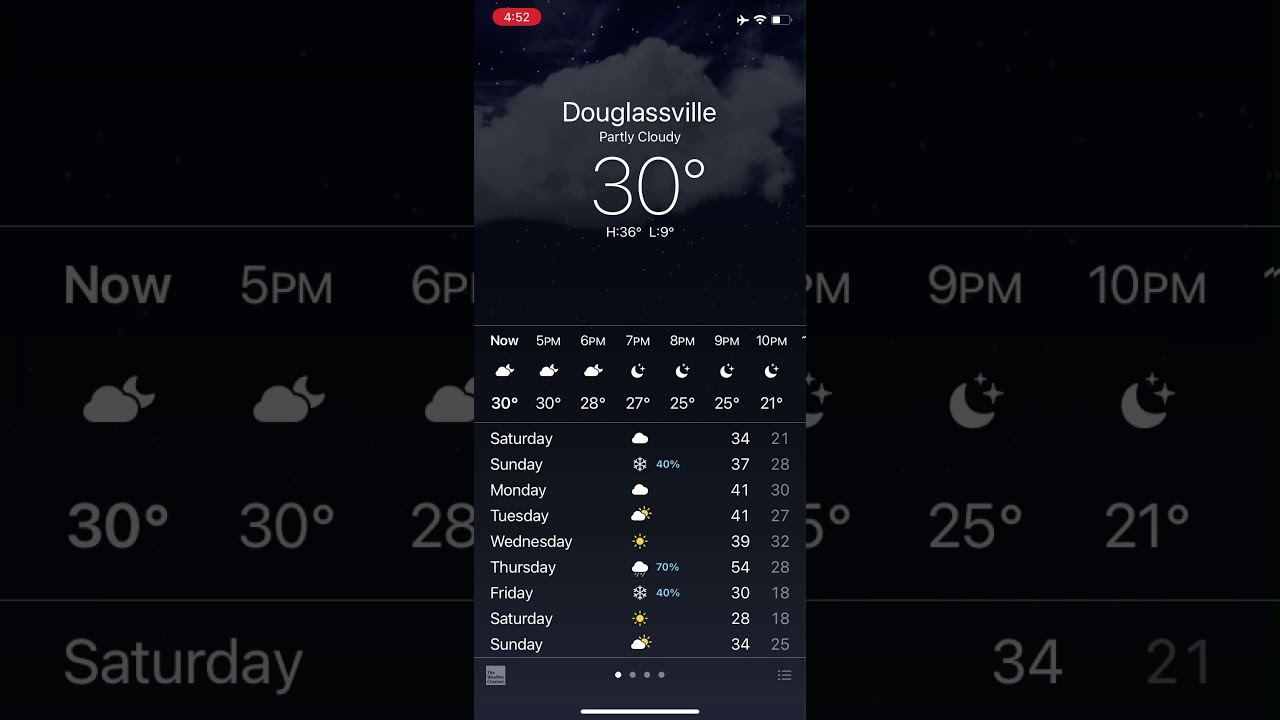The image features weather information displayed against a black background with white text. At the center, within a red box, the time is shown as "4:52" in white text. To the right, several icons are depicted: an airplane, a Wi-Fi signal, and a half-full battery.

The main focus of the display is the weather forecast for Douglasville, where the current condition is partly cloudy with a temperature of 30°F. The day’s high is expected to be 36°F, while the low is forecasted at 9°F. 

Below this, an hourly breakdown indicates:
- 30°F at 5 p.m.
- 28°F at 6 p.m.
- 27°F at 7 p.m.
- 25°F at 8 p.m.
- 25°F at 9 p.m.
- 21°F at 10 p.m.

The extended forecast for the week is as follows:
- **Saturday:** High of 34°F, low of 21°F, cloudy.
- **Sunday:** Snow with a 40% chance, high of 37°F, low of 28°F.
- **Monday:** Cloudy, high of 41°F, low of 30°F.
- **Tuesday:** Partly cloudy, high of 41°F, low of 27°F.
- **Wednesday:** Sunny, high of 39°F, low of 32°F.
- **Thursday:** 70% chance of rain, high of 54°F, low of 28°F.
- **Friday:** 40% chance of snow, high of 30°F, low of 18°F.